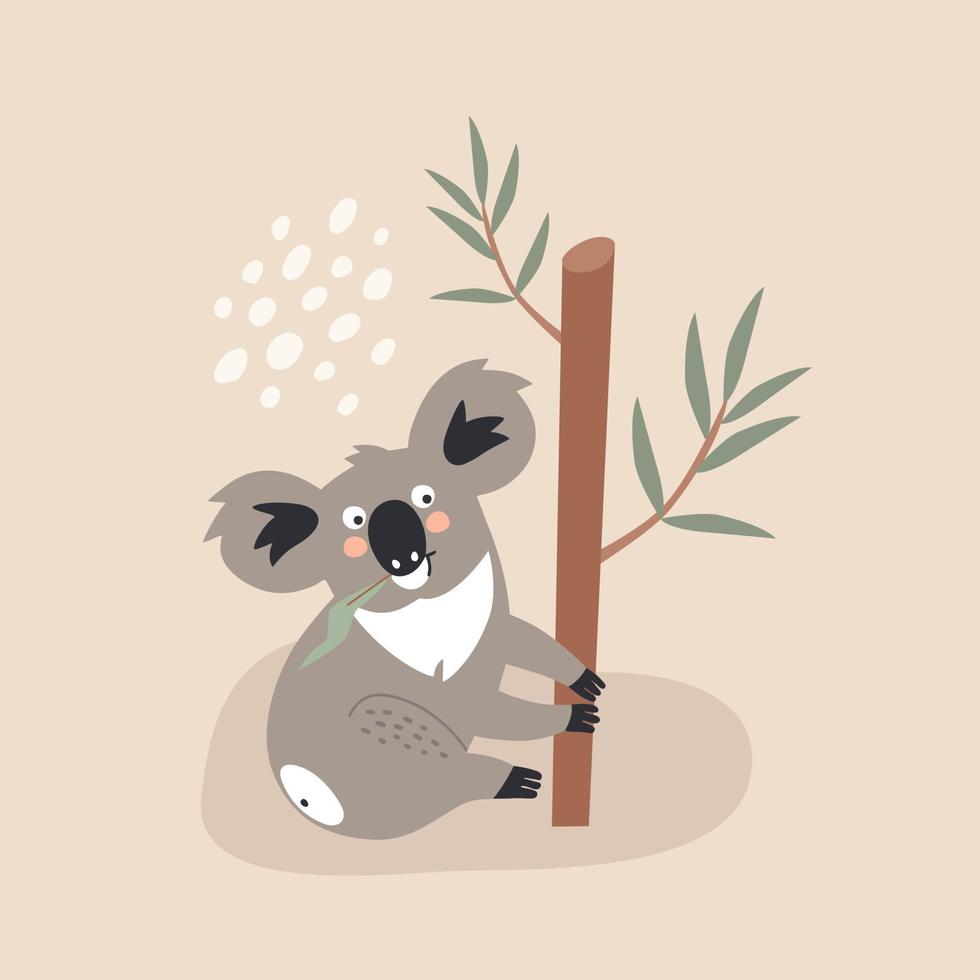This is a colorful flat-design illustration of a koala clinging to a tree branch that has been cut off at the top. The koala, predominantly gray with white patches on its chest, lower mouth, and one leg, has black feet and a black nose with white nostrils. Its claws are long and black, gripping the branch determinedly. The koala's ears are gray with black fur on the insides, and its eyes are wide open, with black pupils in white sclera, giving it a somewhat startled expression. Rosy pink blush marks accentuate its cheeks beneath its eyes. A green leaf is tucked in its smiling mouth, adding a playful touch to the scene. The background of the illustration is a soft lavender color, enhancing the whimsical feel of the artwork. Detailed and vivid, the drawing showcases three of the koala's legs visibly, with the fourth leg partially hidden behind it, creating a charming, albeit slightly eerie, character study.